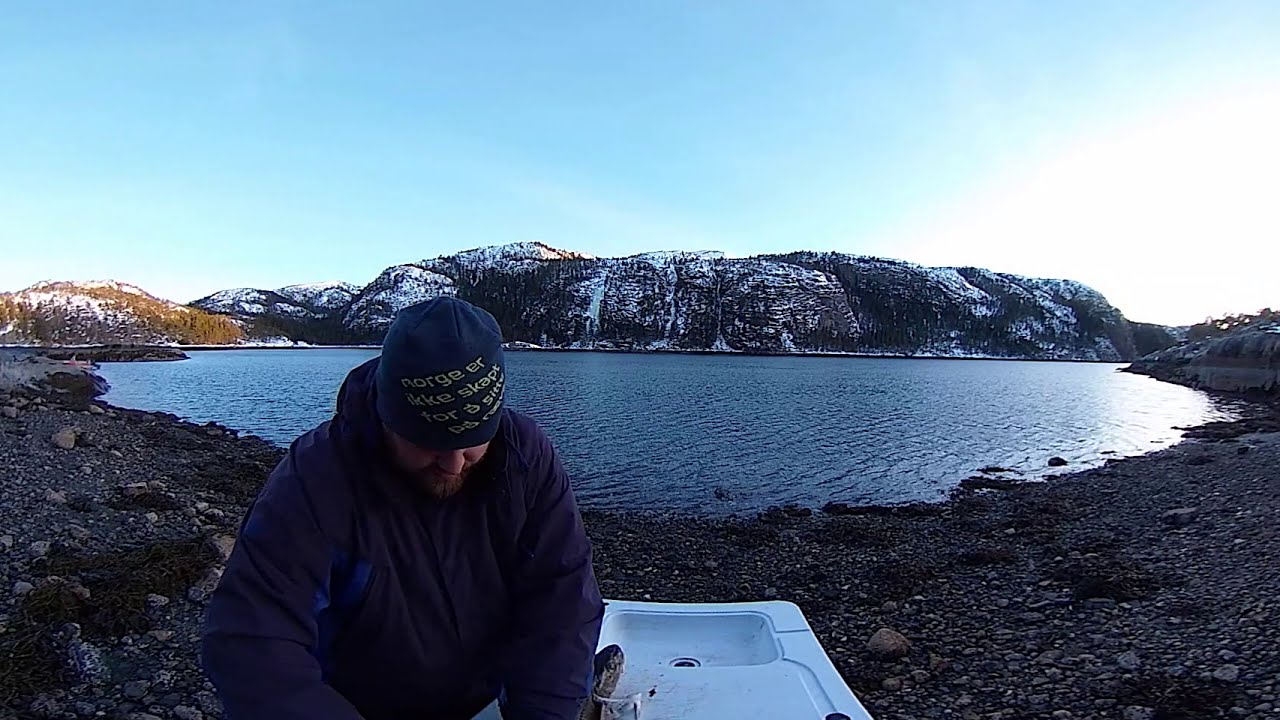In this color panoramic photograph, a man stands slightly to the left of center, wearing a dark navy hooded sweatshirt under a blue coat and a beanie cap with illegible white script. He has a beard and his head is tilted forward, obscuring his face. Surrounding him is a rugged, cold landscape under a partly cloudy sky. In the distance, snow-covered mountains with scattered trees reach towards a horizon lined with a blend of darker and lighter hills. A vivid, blue lake spans the width of the image, bordered by a mix of small rocks and dirt in the foreground. Prominently featured next to the man is a white, camp-style sink with a drain. While his exact activity is unclear, he seems engaged with something at the sink, possibly washing off an object, potentially a fish. The scene captures a solitary moment of outdoor activity against a striking natural backdrop.